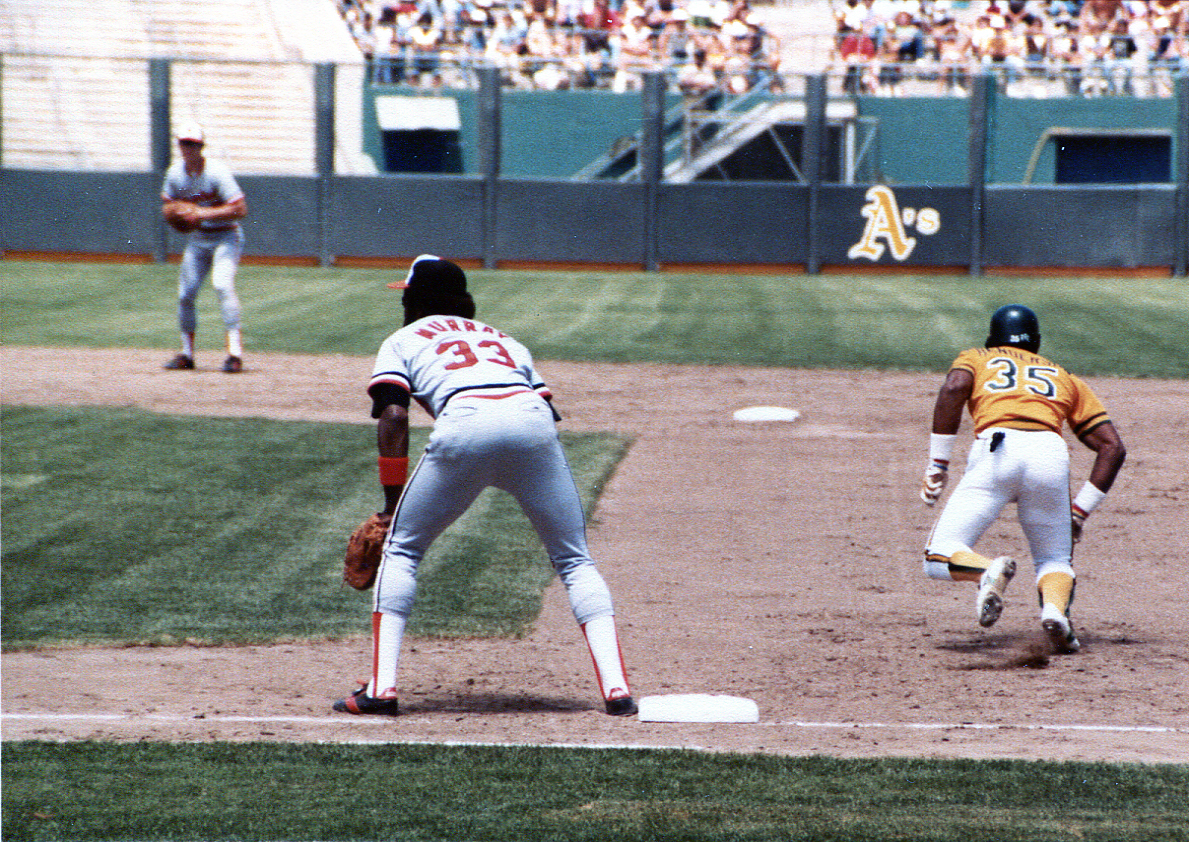The image captures a vibrant scene of a minor league baseball game on a lush, dark green field. The Houston A's or New York A's, known more familiarly as the Oakland A's, appear to be playing in their home stadium, evidenced by the signage featuring the possessive 'A's' in gold near the bleachers and fencing.

In the foreground, positioned along the first baseline, player number 35 from the yellow team, dressed in a gold jersey, white pants, and yellow socks, is seen sprinting between first and second base, attempting to steal a base. He wears a black batting helmet and white batting gloves, kicking up dirt as he races.

Defending against the steal, number 33, named Murray, from the opposing team in gray uniforms with red writing, has his back to the camera. He stands with his right foot touching first base, poised to react. Murray has dark skin and a red armband wrapped around his forearm, and he’s equipped with a baseball glove on his left hand. Further down the field, another gray-uniformed player with a baseball glove holds a defensive stance near where second and third bases are positioned, ready to assist in the play.

The stadium's closely-mowed grass contrasts sharply with a black segmented wall, and the stands above are filled with out-of-focus spectators eagerly watching the game’s unfolding drama.